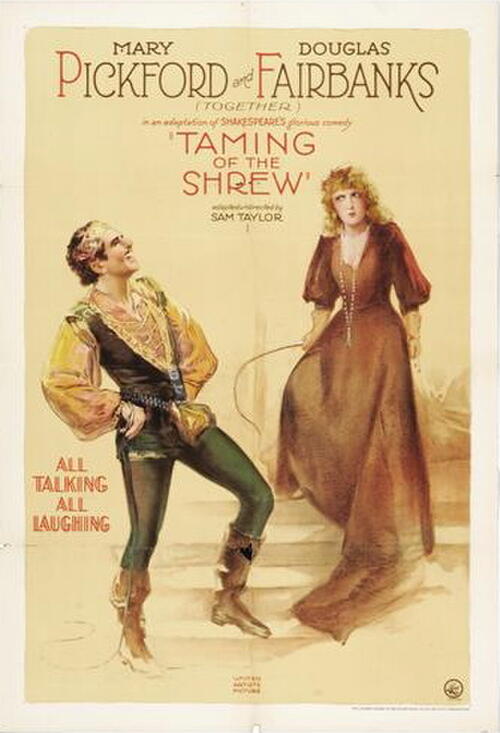The image is a vintage poster promoting an adaptation of Shakespeare's comedy, "The Taming of the Shrew," featuring Mary Pickford and Douglas Fairbanks. The color scheme consists of a light yellow background with orange and tan accents. At the top of the poster, it prominently reads "Mary Pickford and Douglas Fairbanks Together," followed by smaller text indicating "Shakespeare's Taming of the Shrew" and the name "Sam Taylor." In the lower left corner, the tagline "All Talking, All Laughing" is displayed. The artwork depicts Douglas Fairbanks standing on a staircase, wearing green tights tucked into brown boots, a green-brown vest with yellow and orange puffy sleeves, and a gold headpiece. He is leaning back with a laughing expression, hands on hips. Next to him, Mary Pickford is seen in a floor-length red dress with puffy sleeves and a necklace, her curly hair cascading over her shoulders. She holds a whip in one hand and looks visibly disgruntled and angry, adding to the comedic tension portrayed in the scene.